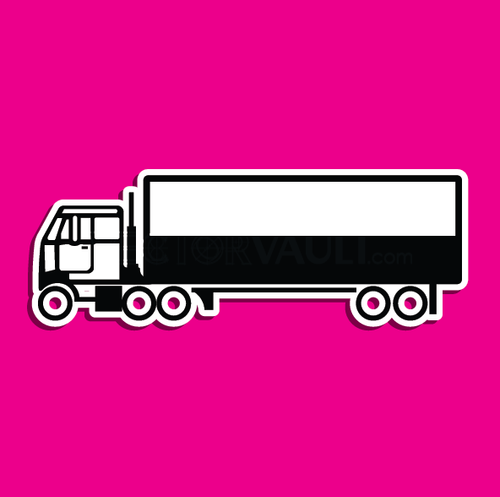The image features a digital or animated icon of a semi-tractor trailer truck set against a solid dark pink square background, which slightly lightens towards the top. The truck, centrally positioned and facing left, is depicted in a cartoonish style. Its cab is a vertical rectangle with an angled windshield, colored in black and white, and includes a prominent side view mirror and a vertical black exhaust pipe behind it. The trailer, a horizontal rectangle, is white on the top half and black on the bottom, with black and white outlining. There are five wheels beneath, with hubs matching the dark pink background and black outlining. This image, likely computer-generated, contains no text and features vivid colors of hot pink, white, black, and accents of gray for shading.